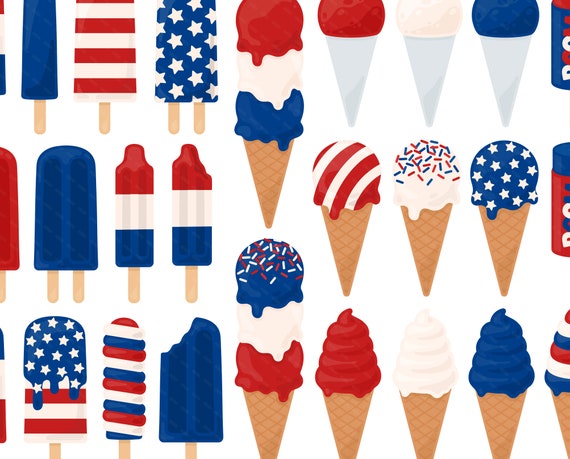This image showcases a series of digitally created, vector clip art illustrations of patriotic-themed ice creams and popsicles, prominently featuring the colors red, white, and blue to symbolize the United States. Set against a white background, the illustrations are arranged in three horizontal rows.

In the first row, you can see a variety of popsicles including a blue one, a red-and-white striped one, and a blue popsicle adorned with white stars. There are also ice cream cones with scoops in patterns like a triple-scoop with red, white, and blue scoops on a gray cone, a red scoop on a blue cone, and combinations with white and blue. The edge of a red, white, and blue can is also visible.

The second row displays more popsicles such as a double red one, a blue fudgsicle-type twin-stick variety, and cylindrical red, white, and blue lollipops. Among these are ice cream cones featuring vanilla with sprinkles, blue backgrounds with white stars, and red-and-white striped motifs—all on brown cones. Additionally, there are swirled red, white, and blue popsicles, a blue fudgsicle with a bite taken out, and soft serve cones in patriotic colors.

The last row continues the theme with soft serve ice cream cones in red, white, blue, and combinations of these colors on brown cones.

Each illustration meticulously uses color and design to evoke a sense of patriotism without the use of any text, making for a vibrant and festive collection of ice cream images.